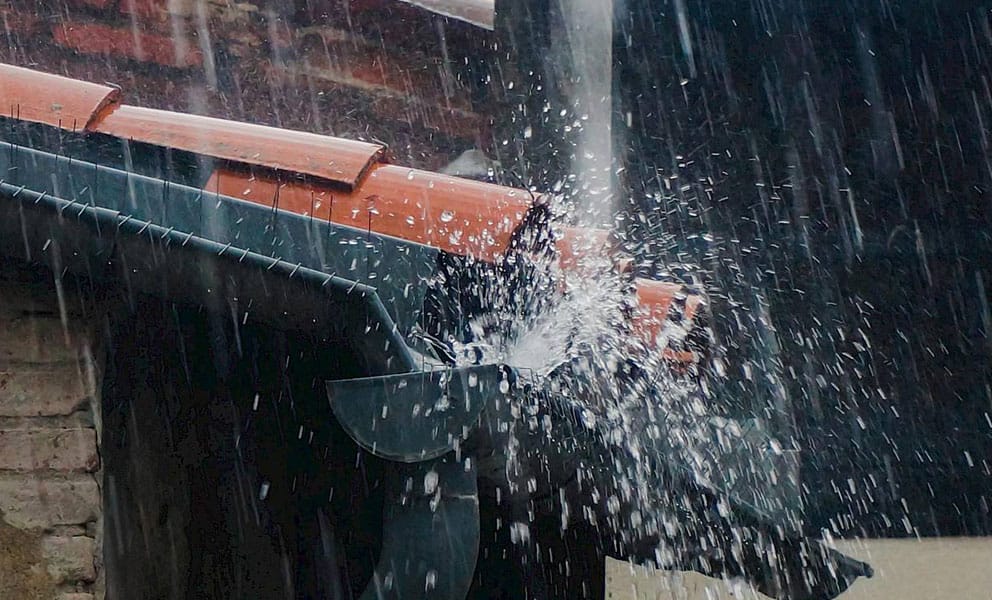This photograph, taken during rainfall, captures the dynamic interaction of water with the black rain gutters attached to a building. The gutters form a zigzag pattern, with one extending from the upper left corner and the other from the center towards the bottom right, converging at the midpoint where a dramatic splash occurs. The rainwater from the left gutter collides with the water in the lower gutter, creating a vivid splash effect. The image also features a segmented view of the environment: a tan, partially visible brick wall on the lower left, and red roof shingles. The background is predominantly black, likely due to shadows, which provides a striking contrast to the splattering water droplets and the rain streaks further evidenced on the right side of the image. The damp atmosphere of the scene, marked by the wet red roof and the blurred water droplets, perfectly encapsulates the essence of a rainy day.